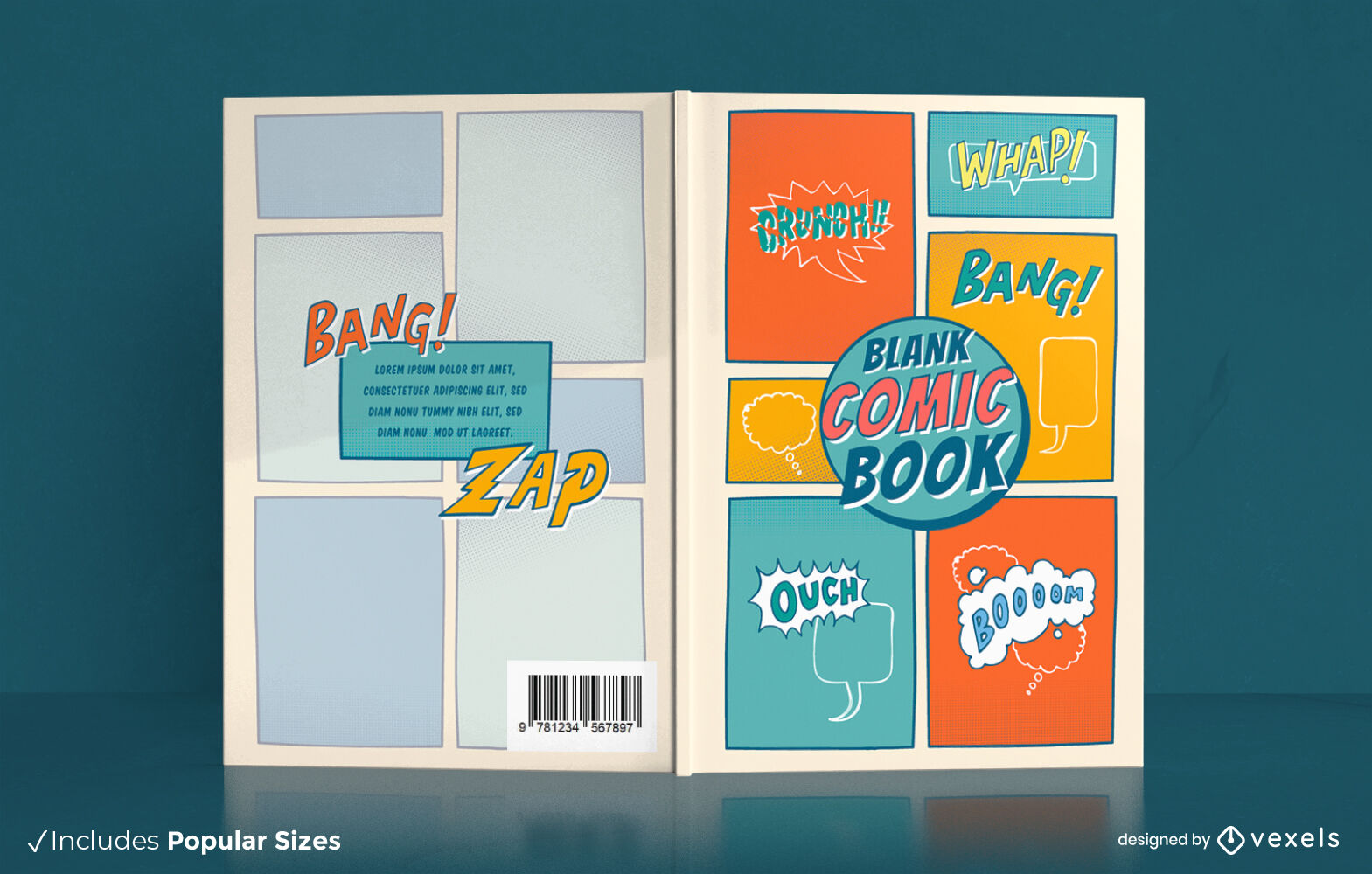The image showcases a blank comic book displayed against a solid bluish-teal background. The comic book is open, revealing both the front and back covers. The front cover is vibrant, featuring a mix of orange, blue, and yellow colors with various action panel windows containing words like "crunch," "whap," "bang," "ouch," "boom," and "zap" in bold, comic book-style text. At the center of the front cover, there is a circle containing the title "Blank Comic Book." The back cover includes text "Lorem Ipsum, Dolor, Sit Amet, Consecutor, Adepson, Elite," which appears to be placeholder text, as well as action words like "Bang" in red and "Zap" in yellow. A barcode is located at the bottom with the numbers 9 7 8 1 2 3 4 5 6 7 8 9 7. In the bottom left corner of the cover, there's a checkmark with the label "Includes Popular Sizes," and in the bottom right corner, it states "Designed by Vexels." The comic book lacks characters or an actual story, emphasizing its function as a customizable template.